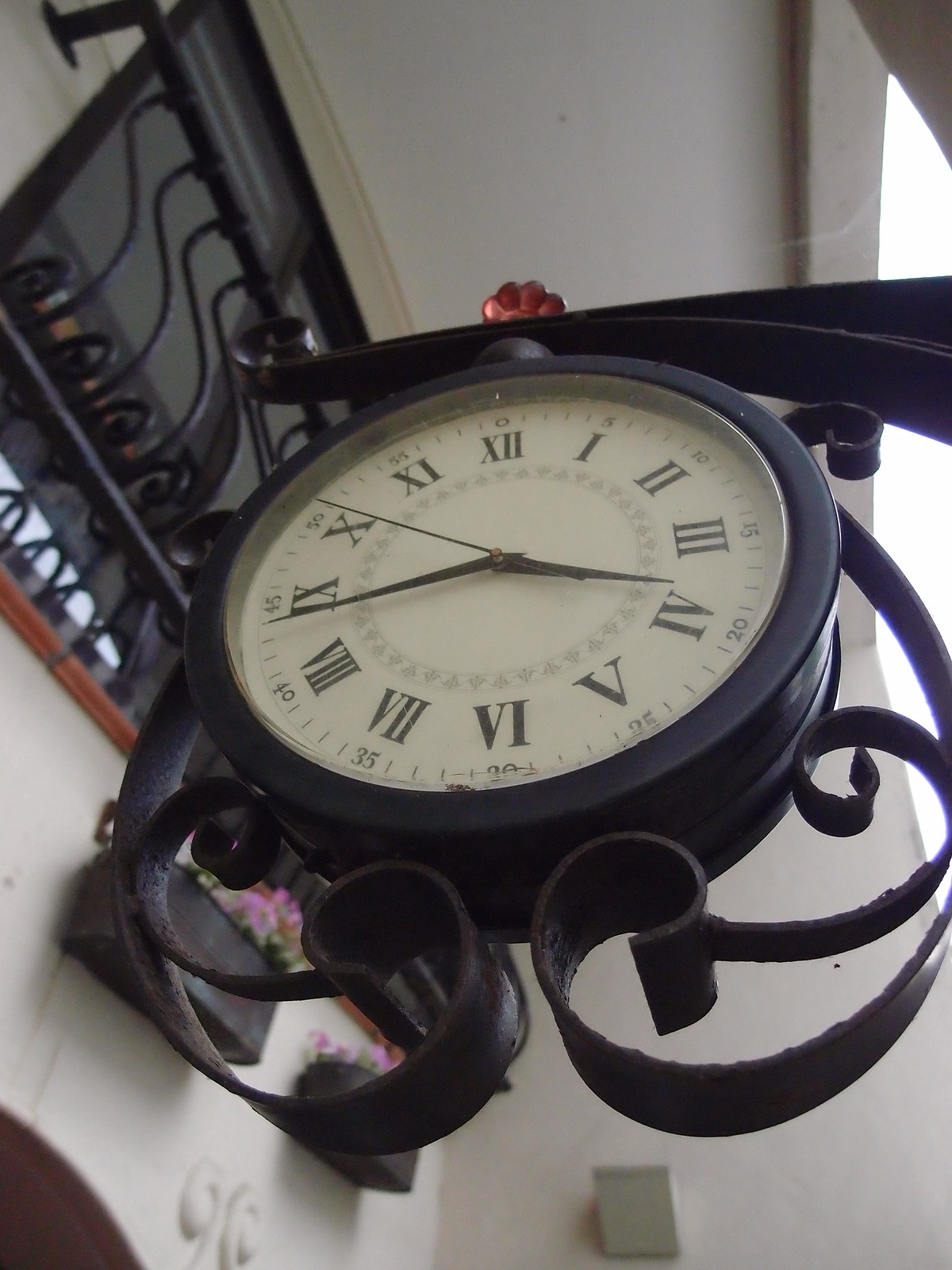This image features a close-up of an intricately designed iron clock suspended from a wall within an unidentified building. The clock boasts detailed iron craftsmanship, with elegant swirling patterns and paisley motifs adorning either side. These swirls extend from the clock's base, curling inward, while additional paisley designs arch upwards, framing the clock. A red flower petal is visible, partially protruding from the top of the clock, resting on an iron bar that extends horizontally from the wall. This bar also curls at its end, forming a loop above the clock. In the bottom left corner of the image, the upper part of an archway is visible, accompanied by a cement or possibly sculpted embellishment to its right. Additional ironwork is present above the clock, consisting of three angled sections with an 'S' curve and curled ends, enhancing the image's architectural elegance.